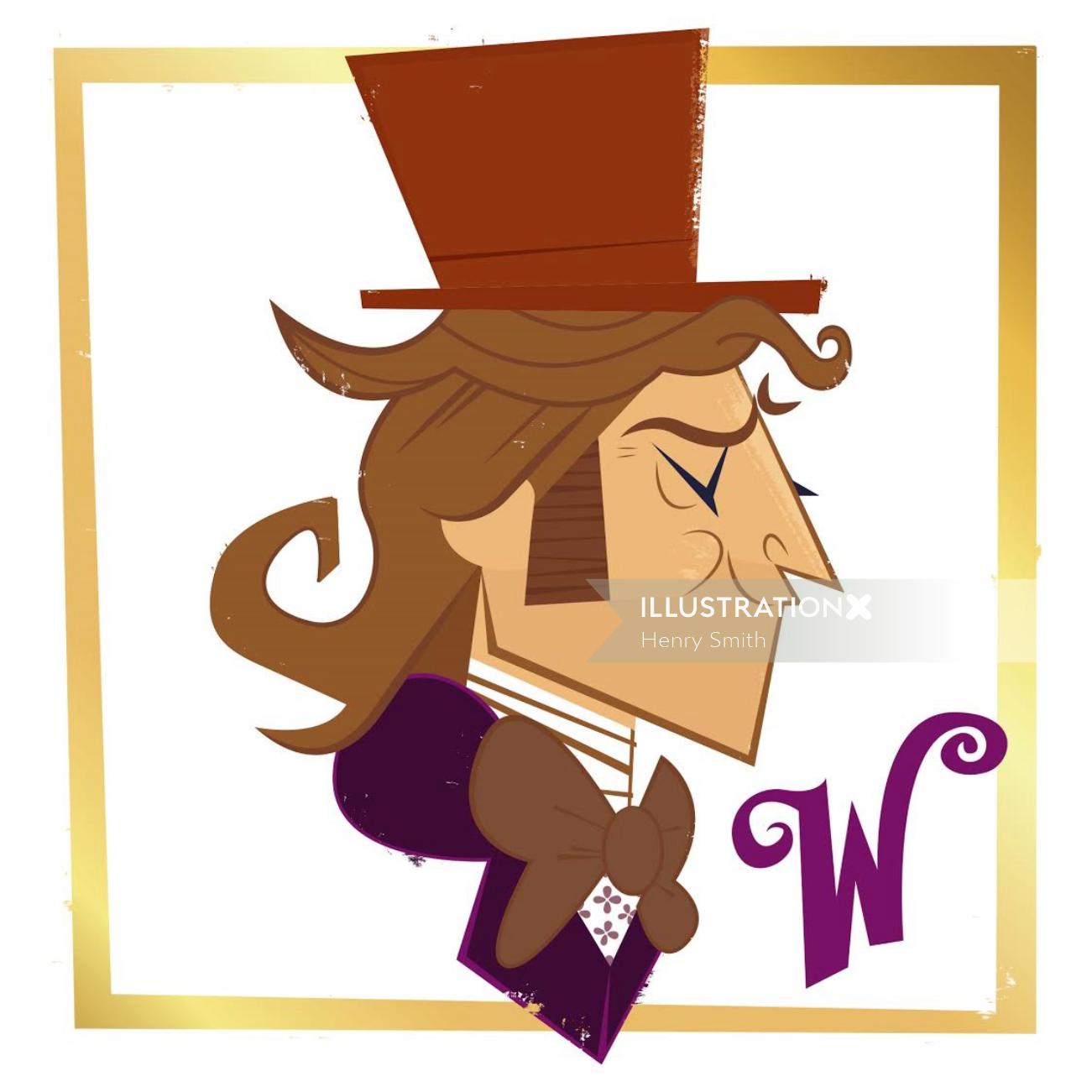This is a stylized digital illustration of Willy Wonka, credited to Henry Smith as shown in the watermark on the right-hand side of the image. The artwork features a side profile view of Wonka, who is facing to the right with a smirk on his face and his eyes closed. He wears a rusty brown top hat, a large light brown bow tie, and a royal purple coat. His long wavy hair and prominent sideburns are shades of brown, adding to the angular, slightly retro aesthetic reminiscent of the late 60s or early 70s. Beneath the bow tie, he dons a white shirt adorned with purple flowers, and above it, a high white collar with brown stripes. The illustration is completed with a shiny golden border that varies in lightness and darkness and a white background. In the lower right-hand corner is a distinctive purple "W" in the classic Wonka font.